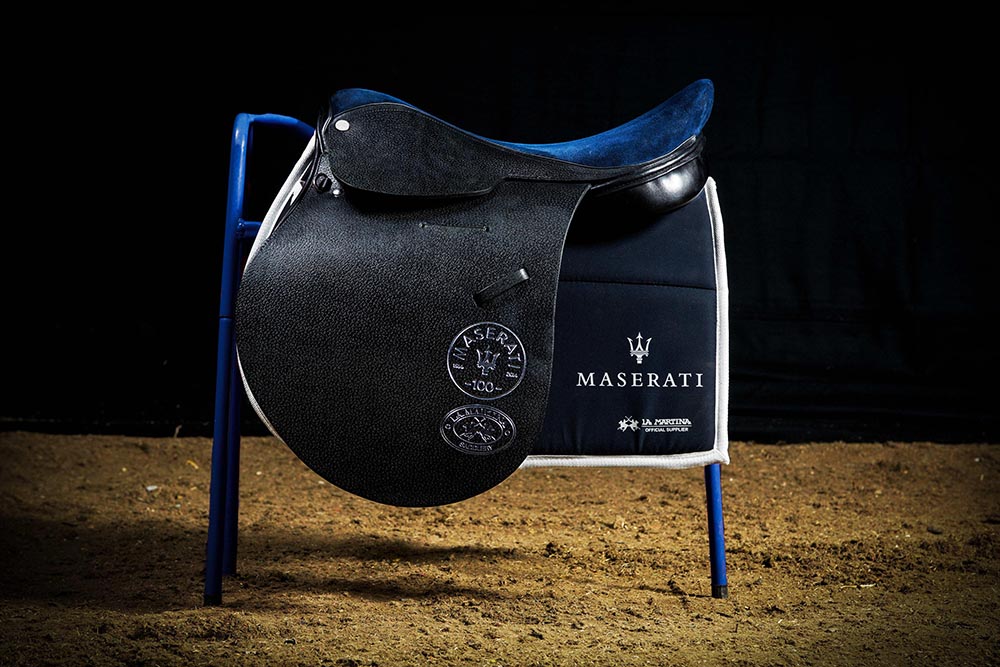The close-up image features a horse saddle positioned centrally against a solid black or dark blue fabric backdrop, with a patch of dry dirt at the bottom. The saddle, which is smooth and light black in color, is mounted atop a blue frame. Beneath the saddle lies a navy blue blanket with white etching. Prominently displayed in the lower right-hand corner, the word "Maserati" appears in white letters, accompanied by its emblem, followed by the number "100." A second, unreadable circle is positioned below this emblem. The overall composition and details suggest a professional product photograph that might be showcased on a company website for promotional purposes. The color palette is predominantly black, white, gray, and different shades of brown.